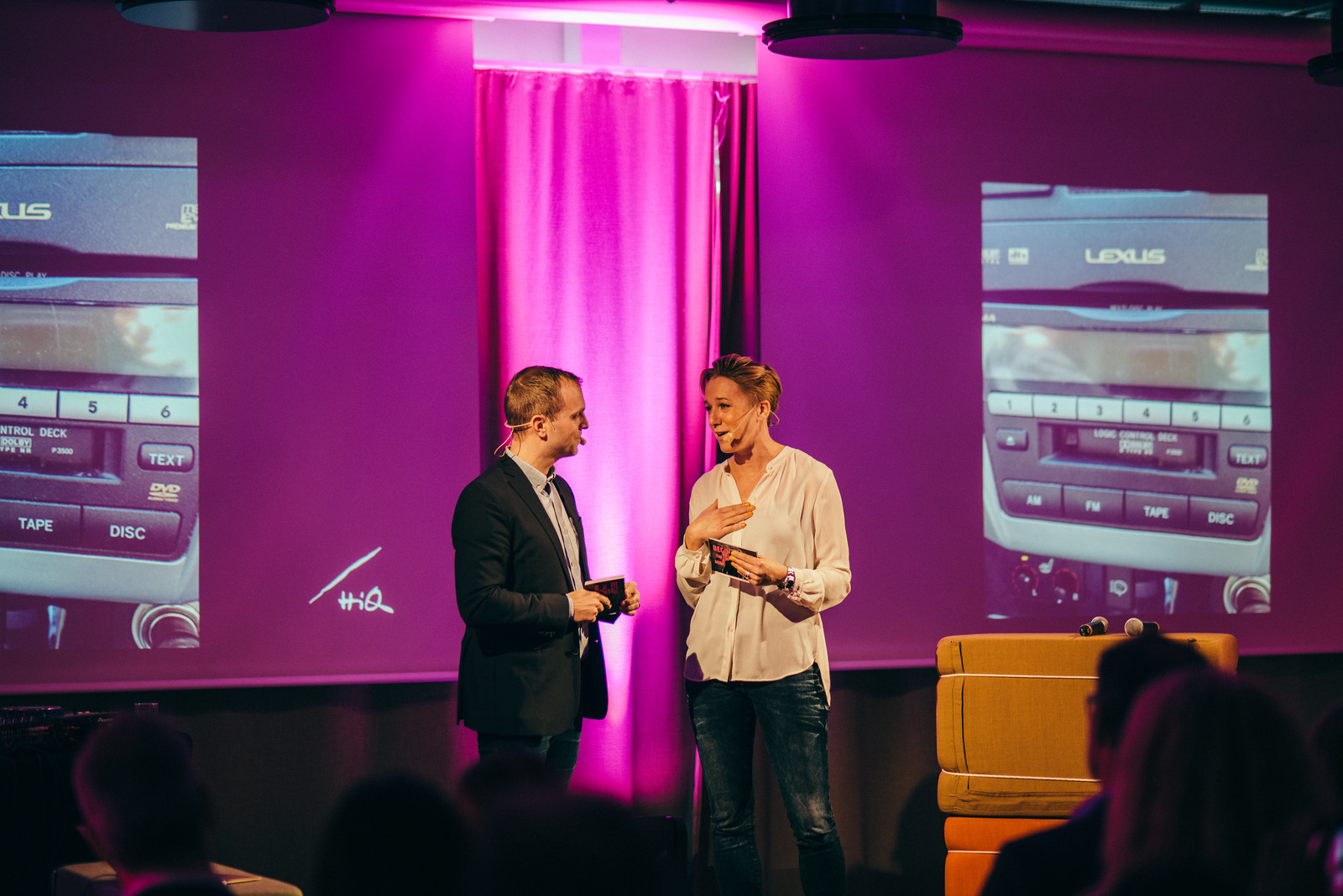In this image, two presenters are standing on a stage in front of a seated audience, delivering a presentation on behalf of Lexus. The background features illuminated purple projector screens displaying images of a Lexus stereo system, including a CD player and contemporary radio dials, bordered by a rich purple curtain. The woman on the right, who has brown hair, is dressed in denim jeans and a white long-sleeve blouse, and she holds index cards as she addresses the audience. The man to her left, also with brown hair, is wearing a black suit jacket, a gray shirt underneath, and jeans. Both presenters are equipped with headsets for clear communication. A podium is visible to the left, framing the scene, which highlights the modern Lexus technology they are discussing.